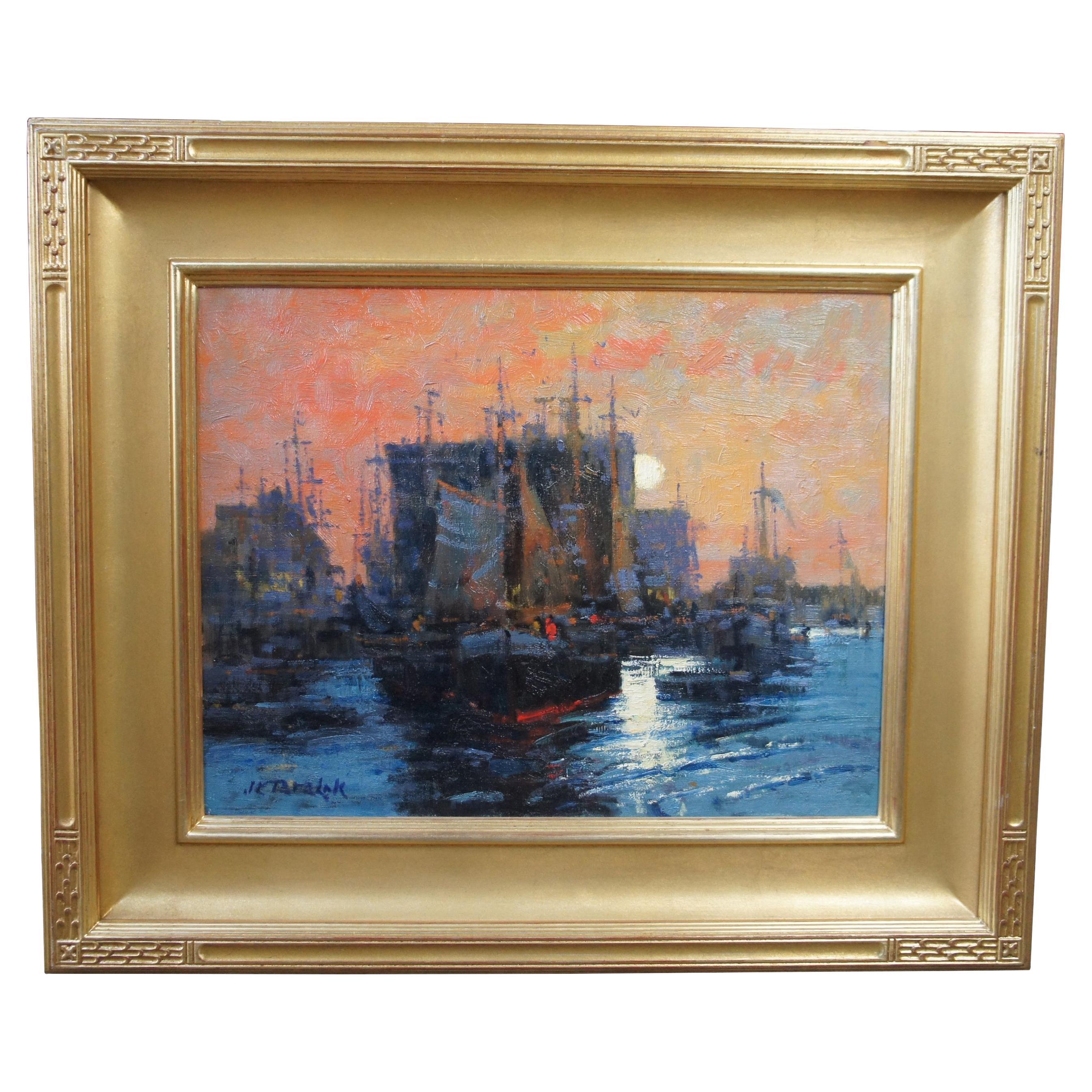The image shows a vintage-style painting, likely oil-painted, surrounded by a thick, ornate, rose-gold frame that measures about two to three inches in width. The frame features intricate patterns at each of its four corners, highlighting its classical design. The painting itself depicts a bustling harbor scene at dusk or dawn, with the sky bathed in a mesmerizing blend of pink, orange, blue, and purple hues. The water beneath the ships is a deeply rippled blue, capturing the serene yet dynamic nature of the sea. The harbor is populated with a fleet of ships reminiscent of English vessels from the 1700s or 1800s, their dark bodies contrasting with striking sails in shades of dark yellow, orange, white, and blue. The setting sun casts a warm glow over the scene, accentuating the historical and picturesque ambiance of the painting. The piece appears to be displayed in a gallery, set against a simple white wall, which further emphasizes the painting's rich details and elegant framing.